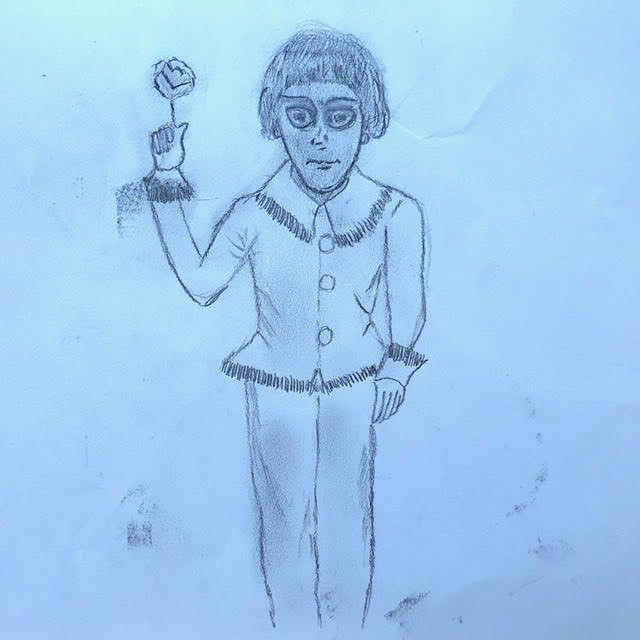The image is a detailed pencil drawing on light bluish paper with darker splotches as part of the background. The drawing depicts a figure with a bowl-cut hairstyle, large eyes, thin arched eyebrows, and a closed mouth, suggesting a contemplative or neutral expression. The person is dressed in a long-sleeved, buttoned-up shirt featuring three prominent buttons and adorned with frilly details at the collar, sleeves, and bottom edge. The attire includes long pants that continue down towards the ankles, where the illustration cuts off, though the pants are less emphasized than the shirt. The figure's right arm is raised, holding a flower that appears to be a rose, though it is not detailed enough to confirm definitively. The left arm hangs naturally by their side. The person, possibly depicted as a little man, might also be wearing earrings, adding to the ornamental nature of the drawing. The entire figure is rendered in shades of light blue with some nuanced facial shading to enhance depth.